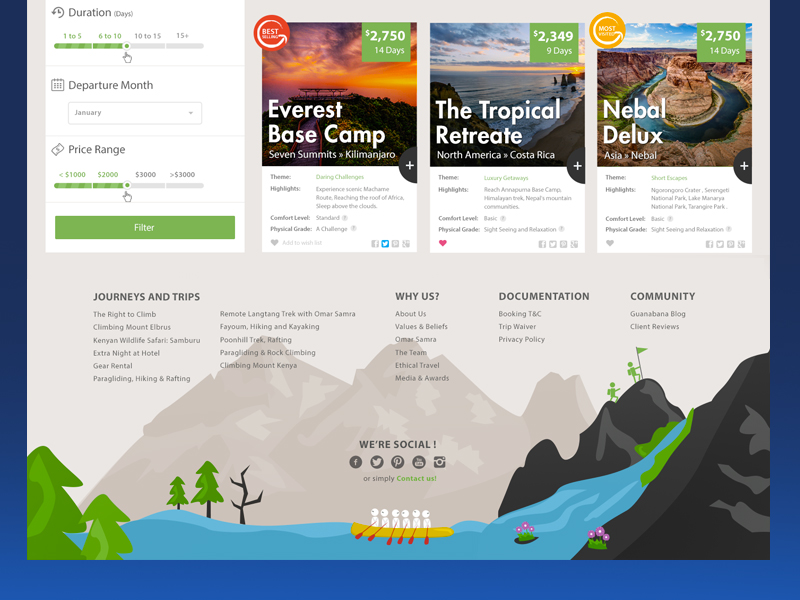**Discover Your Next Adventure on Our Travel Site**

Explore the best travel experiences tailored to your needs. Our easy-to-use website allows you to filter trips based on various parameters, including duration (6 to 10 days), departure month (January), and price range (up to $2000).

Highlighted Options:
1. **Everest Base Camp**:
   - **Category**: Best
   - **Duration**: 14 days
   - **Price**: $2750
   
2. **Tropical Retreat, Costa Rica**:
   - **Category**: North America
   - **Duration**: 9 days
   - **Price**: $2300
   
3. **Nepal Deluxe**:
   - **Category**: Asia
   - **Duration**: 14 days
   - **Price**: $2750

At the bottom of the page, you’ll find sections including **Journeys and Trips**, **Why Us?**, **Documentation**, and **Community**. The site also features charming illustrations of mountains, streams, and people canoeing, adding a delightful touch with little flowers.

Stay connected with us on social media through our Facebook, Twitter, and Pinterest links, or simply contact us for more information. The imagery also showcases climbers with a flag at the peak of a mountain, embodying the spirit of adventure that we offer.

**We're Social**: Join our community and start your journey today!